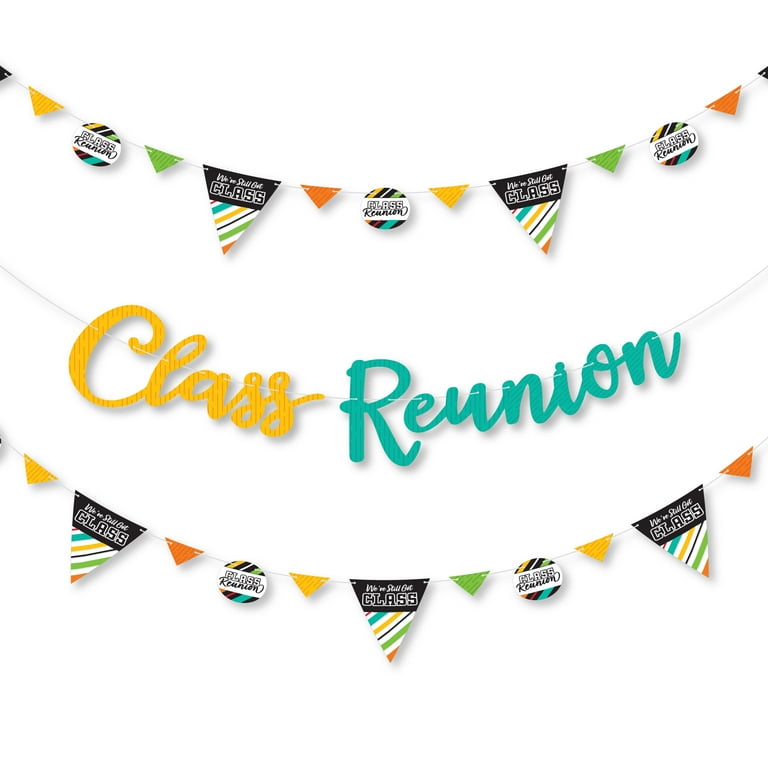The image depicts three festive banners draping from left to right, creating a lively and celebratory atmosphere. The top and bottom banners feature alternating triangular and circular pennants in vibrant colors, including yellow, green, and orange. These pendants bear a mix of black and white text with some of them displaying messages such as "Class Reunion" and "I've Still Got Class" against a multicolored striped pattern background. In the center, the focal point of the display, is a banner with the words "Class Reunion" written in an elegant cursive font—"Class" in a dark yellow hue and "Reunion" in dark turquoise. All three banners are strung on white strings and stand out clearly on a plain white background, giving the impression of being ready to adorn a party or celebration space.